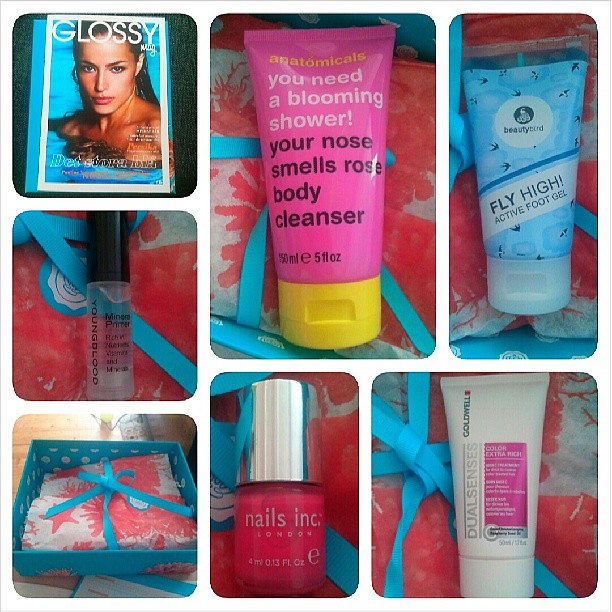The image is a collage of seven photographs showcasing different products. The top-left photo features a seductive woman in a pool on the cover of a magazine named "Glossy." Right below this, there is a spray bottle labeled "Mineral Primer" from Youngblood. Beneath the spray bottle, an open blue box with white dots reveals a coral-patterned blanket inside. At the center-top of the collage, a pink lotion bottle reads "Anatomicals: You Need a Blooming Shower, Your Nose Smells Rose Body Cleanser." To its right, a blue tube named "Fly High Active Foot Gel" is visible. Below these two, a bottle of red nail polish from Nails Inc. is placed next to a white bottle labeled "Dual Senses Color Extra Rich." This collage appears to depict a curated collection of beauty and personal care products, possibly as part of a gift package.